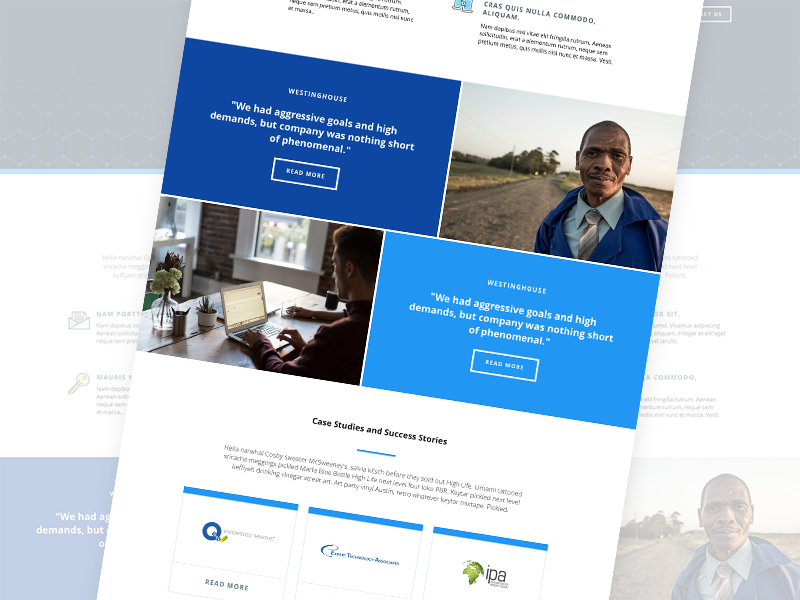The image is a screenshot from a website displaying a pop-up message. The website's interface can be seen in the background, though it's partially obscured by the pop-up, which is tilted at an unusual angle. The centerpiece of the pop-up features a photograph of an African man dressed formally in a collared shirt, tie, and what appears to be an overcoat. Accompanying this image, a blue text box contains the quote: "We had aggressive goals and high demands, but the company was nothing short of phenomenal." Written in a slightly lighter blue box below the main text, the same quote is reiterated. On the right side of the pop-up, there is a secondary image of a Caucasian man focused on typing at a small laptop. The company's name or purpose is not specified within the pop-up or the screenshot.